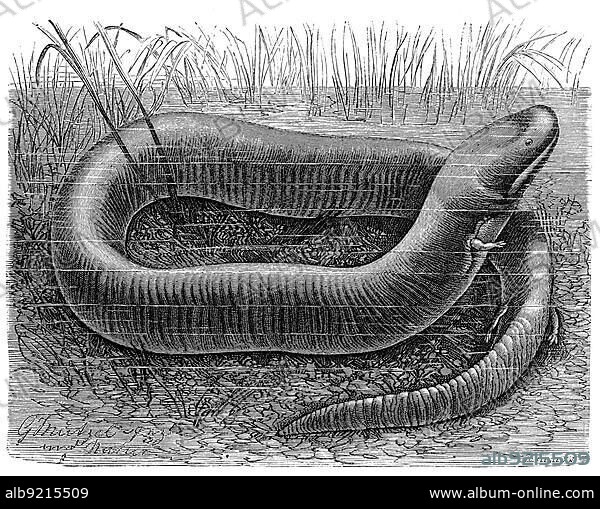The black and white pen and ink drawing depicts a peculiar, elongated creature with a snake-like body, head, and beady eyes. Although its form is reminiscent of a snake, it is distinguished by small arms and legs – one arm is visible from the top portion of its body, while the other is obscured due to the creature's positioning, and the back end has two tiny legs. The creature is coiled, with its head overlapping its body and the tail tapering to a fine point. It is set in a swamp environment, with water visible in the background and plants, possibly seaweed, emerging from the water. The artwork features text, though mostly illegible, except for a website address, "www.album-online.com," in the bottom left-hand corner where there's also a signature.